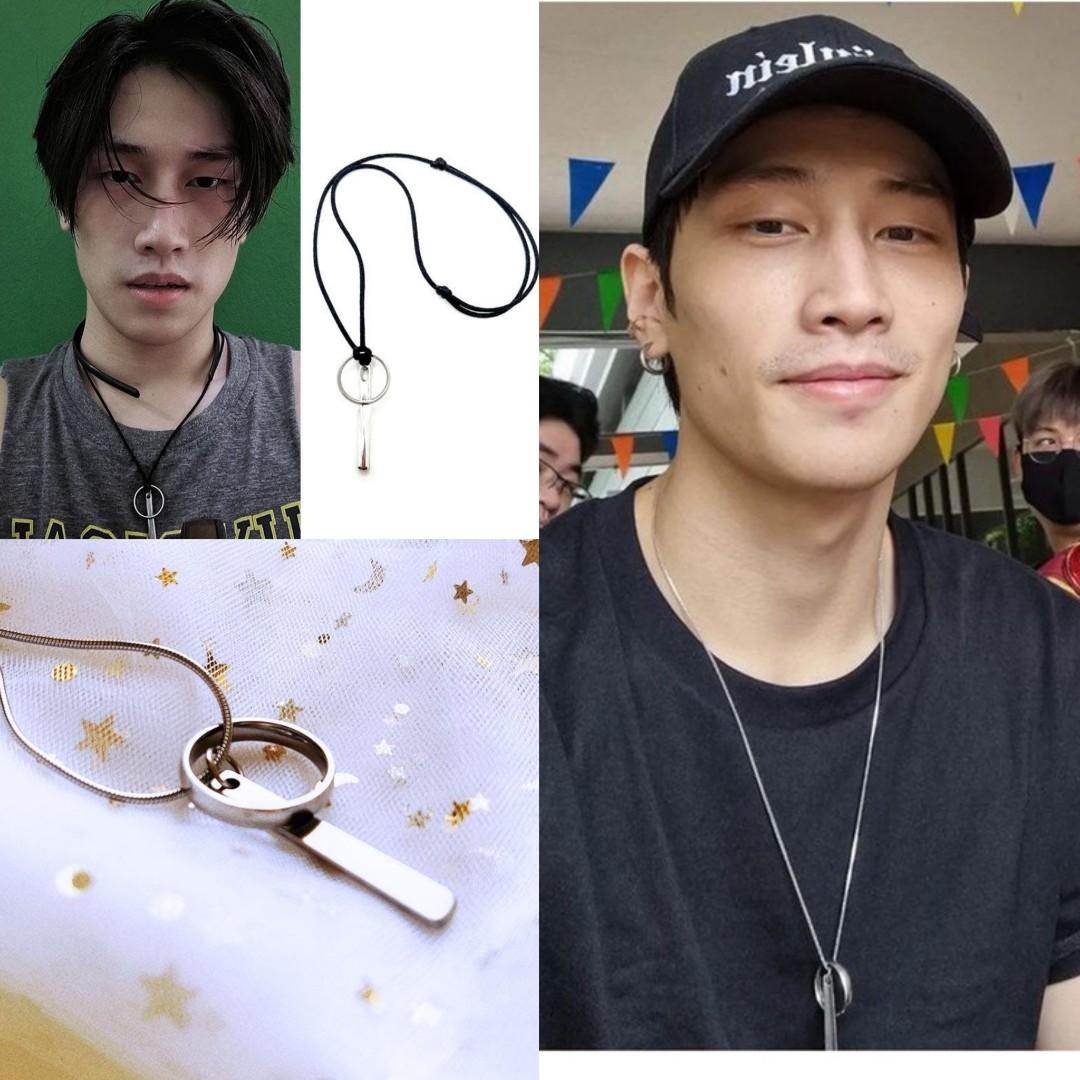The image features a collage of four photographs showcasing an Asian man and a distinctive necklace from multiple angles. In two of the pictures, the young man, appearing to be around 20 years old, is the focal point. In one photo, he dons a black baseball cap, a dark gray T-shirt, and a silver chain necklace that features a simple silver ring, reminiscent of a wedding band, paired with a one-inch rectangular silver bar. He has short hair, an earring, and a neutral expression as he looks straight ahead. In the second image of him, he is without the hat, his shaggier hair falling somewhat into his eyes, and he sports the same necklace pieces but strung on a black cord instead of the silver chain. His expression in this image is more brooding.

The remaining two images focus solely on the necklace itself. One shows the necklace laid against a white background, highlighting its intricate details—the silver ring and the rectangular bar threaded through the chain. The final image presents a close-up of the necklace on a background adorned with gold stars, offering a clearer view of the metallic elements against the textured cloth. This detailed presentation suggests it may be an advertisement for the unique and versatile jewelry piece.